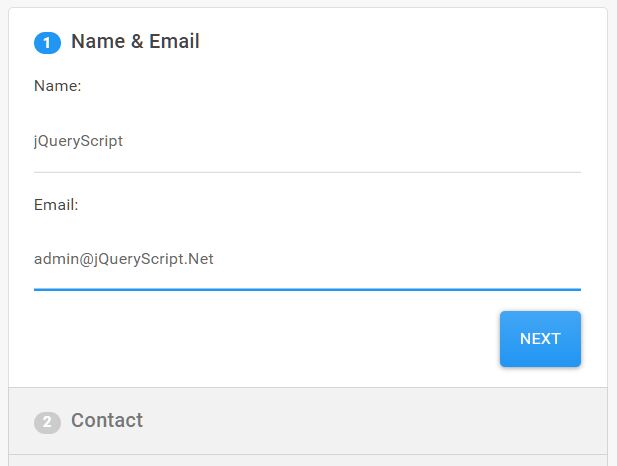The image displays a white box with a gray border surrounding all four sides. The bottom border is significantly taller and thicker than the others. Inside this box, there is a smaller white box containing a blue circle with a white number '1' in the center. To the right of this circle, bold black text reads "Name and Email." Below this heading, in regular text, "Name:" is written, followed by a blank space. 

After skipping a few lines, the text "jQuery Script" appears, followed by another blank line. A light gray horizontal line spans nearly the entire width of the white box, stopping just short of the edges. Below this line, the text "Email:" is displayed, again followed by a blank space. Skipping a couple of lines further, the text "admin@jqueryscript.net" is written, under which another blue line of similar length to the previous one is found. Beneath this line, there's a blue square button labeled "Next."

Below the button, there is a dark gray circle containing the number '2,' adjacent to which the word "Contact" is written.